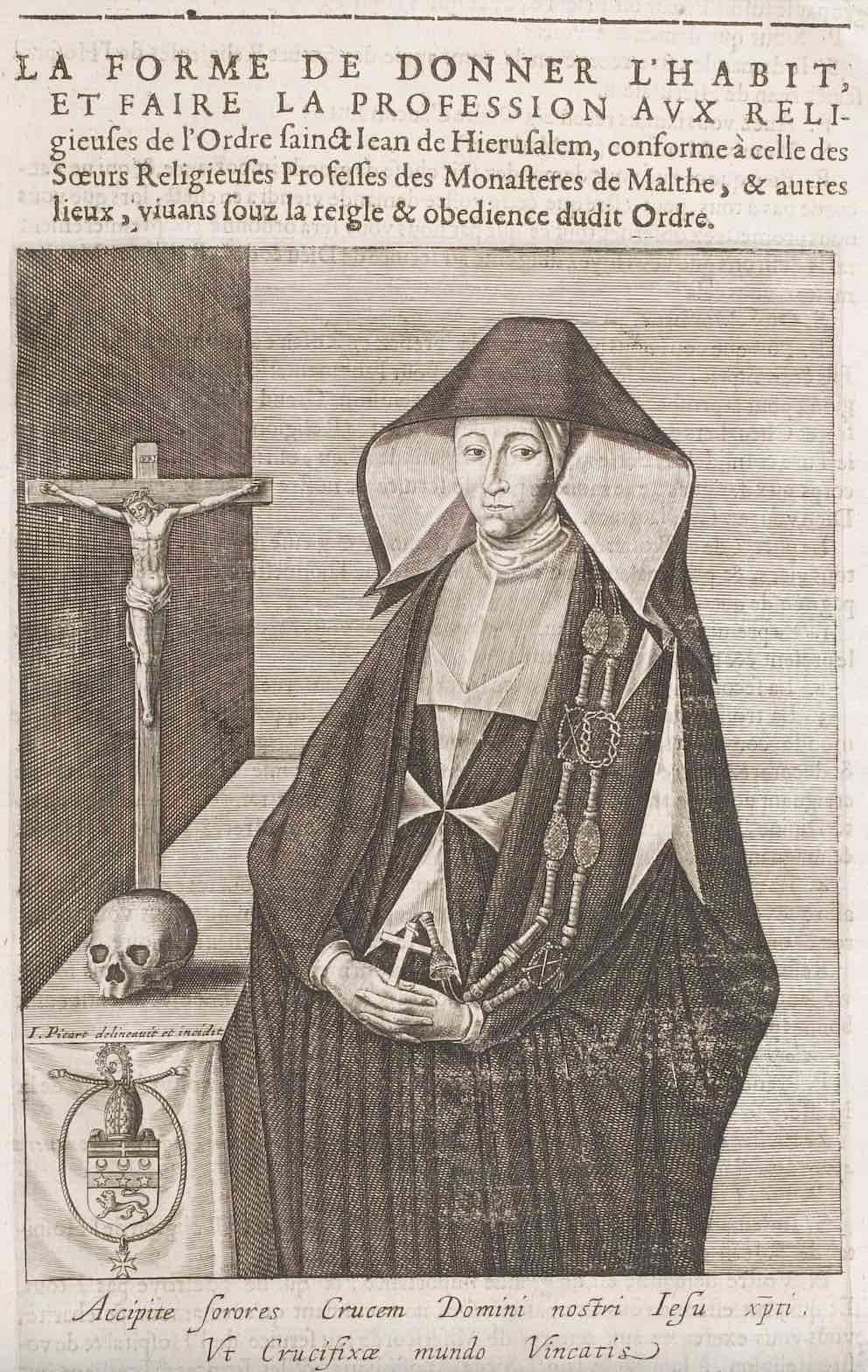The image is a hand-drawn, black-and-white illustration resembling an old newspaper clipping or a book page, in a faded tan color. It depicts a solemn nun, dressed in a traditional habit complete with a wimple and elaborate decorations extending from her neck down to her sleeves. The nun, situated to the right, holds a small crucifix about the size of her hand. 

To the left of the nun stands a crucifix with Jesus, beneath which lies a skull placed on what appears to be a bookshelf-like object draped with a cloth bearing an emblem or coat of arms. The background features a two-toned wall with a gray section behind the nun and a darker, black section behind the crucifix and skull. 

The text above the image, written in French, reads "La Forme de Donner l'Habit et Faire le Professionnel," indicating the guidelines for how a particular order should dress. Below the image and at the bottom of the page, the text appears to be in Latin, though the exact phrases are difficult to discern. The illustration evokes a sense of solemnity and religious devotion, capturing the traditional attire and symbols associated with a nun's profession.